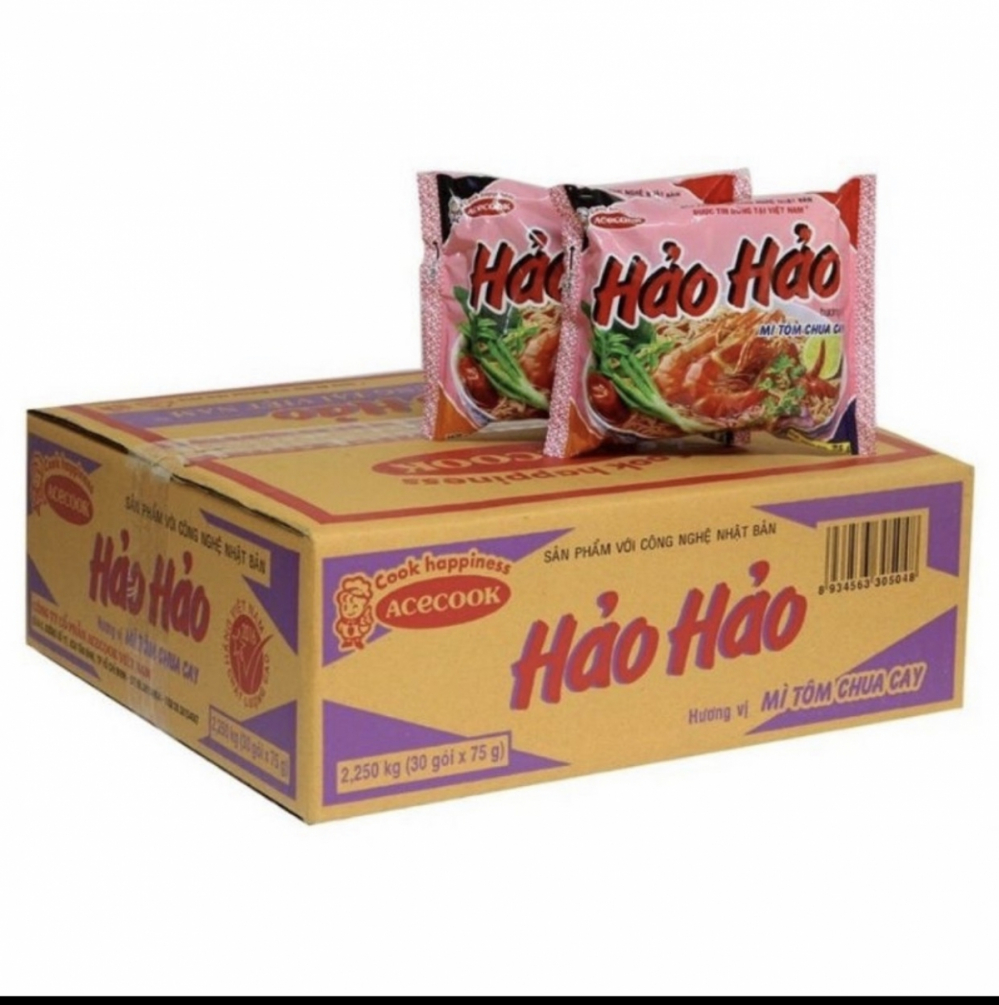In the image, there is a large cardboard box, prominently positioned in the center, taped shut and emblazoned with the text "Cook Happiness Ace Cook" and "Hao Hao" in bold letters. The remainder of the text appears to be in a foreign language, possibly Vietnamese or Thai. The box is primarily purple with accents of red, brown, and possibly green. Resting on top of the box are two smaller packages, which appear to be instant noodles. The color palette of the items includes white, black, tan, red, purple, pink, green, and yellow. The background is stark white, giving the image a clean, minimalist look. A thin black bar runs along the bottom of the image. The overall styling and presentation suggest it is an image designed for a website, perhaps for e-commerce platforms like Amazon or a supermarket website.